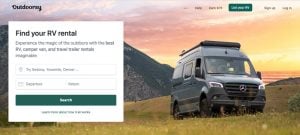This image appears to be a blurry screenshot from an RV rental website, likely Outdoorsy, given the partially readable text at the top. The screenshot itself is notably small and rectangular. The main visual features a large gray and black van parked in a scenic mountainous area with dark greenish-yellow mountain grass. The backdrop showcases a striking pink and yellow sky, suggesting either a sunrise or sunset, with part of a mountain visible to the left of the van. 

A white box with the text “Find your RV rental” is prominently placed over the image, obscuring much of the mountainous background. The box contains additional, unreadable text below, possibly including phrases like "experience the magic of the outdoors with the best RV camper." Additionally, the right side of the image features several placeholders for text, which are unreadable due to the overall blurriness of the screenshot.